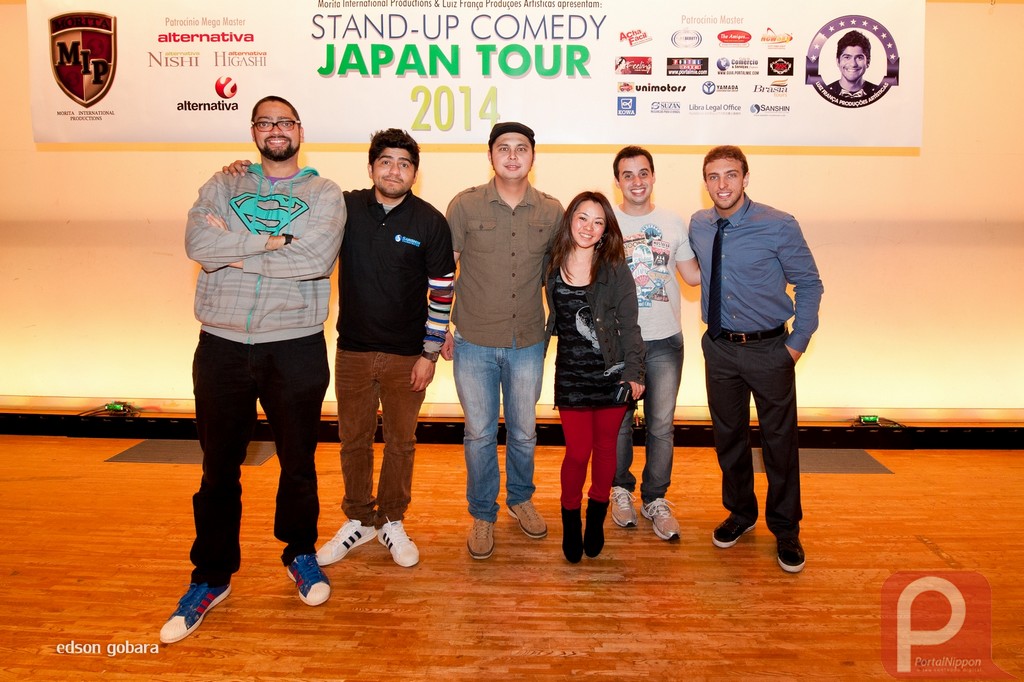In this photograph from the Stand-Up Comedy Japan Tour 2014, six young adults in their 20s to early 30s are posing together, standing on what appears to be the wooden floor of a recreational center. Behind them, a banner emblazoned with "Stand-Up Comedy Japan Tour 2014" is prominently displayed, flanked by various sponsor logos including "Nishi Alternativa." 

The diverse group, consisting of five men and one woman, stands in a relaxed formation, arms around each other's shoulders, all smiling at the camera. Starting from the left, the tallest man sports a grey t-shirt with an aqua Superman logo and has a dark beard and hair. To his right, the second man is dressed in a black polo shirt and brown trousers, with his hair styled in a spiky fashion. 

In the center stands a man in a greenish-brown button-down shirt and jeans, wearing a flat cap. The only woman in the group is fourth from the left, much shorter than her companions, and is wearing a black dress paired with red leggings and an overcoat. To her right, the fifth person is a lighter-skinned man in a graphic t-shirt and jeans. The man on the far right is dressed more formally in a blue button-down shirt and a black tie, complemented by grey slacks.

Additionally, there are two watermarks on the photo: one in the lower left corner that reads, "Edson Gobara," presumably the photographer, and a red "Portal Nippon" watermark in the lower right corner.